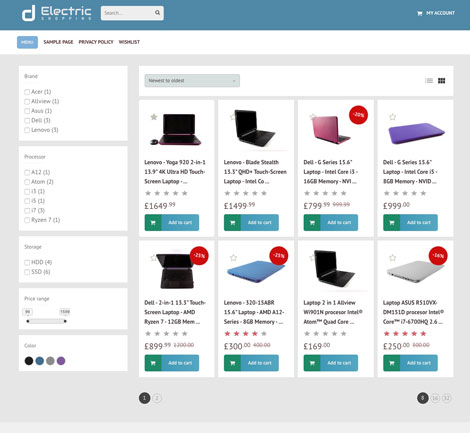This web page from an unspecified website named "Electric [Something]" features a blue border at the top, followed by a search bar and a "My Account" link on the far right. Above the blue border are four navigational tabs, with one currently highlighted.

On the left side of the page, there are several checkboxes presumably for refining search results. To the right of the checkboxes is a dropdown menu. 

The bulk of the page displays eight images of laptop computers, each listed with corresponding prices. The first laptop is black and priced at €1,649.99. The second laptop, also black, is priced at €1,499.99. The third laptop, which is a dark pink color, is available for €799.99. The fourth laptop is purple and priced at €999.99. Another black laptop appears next, priced at €899.99. The sixth laptop is blue and costs €300. The seventh laptop is black and priced at €169, and the final laptop is off-white, costing €250.

Overall, the webpage comprises essential sorting options and a variety of laptop choices, catering to a wide price range.